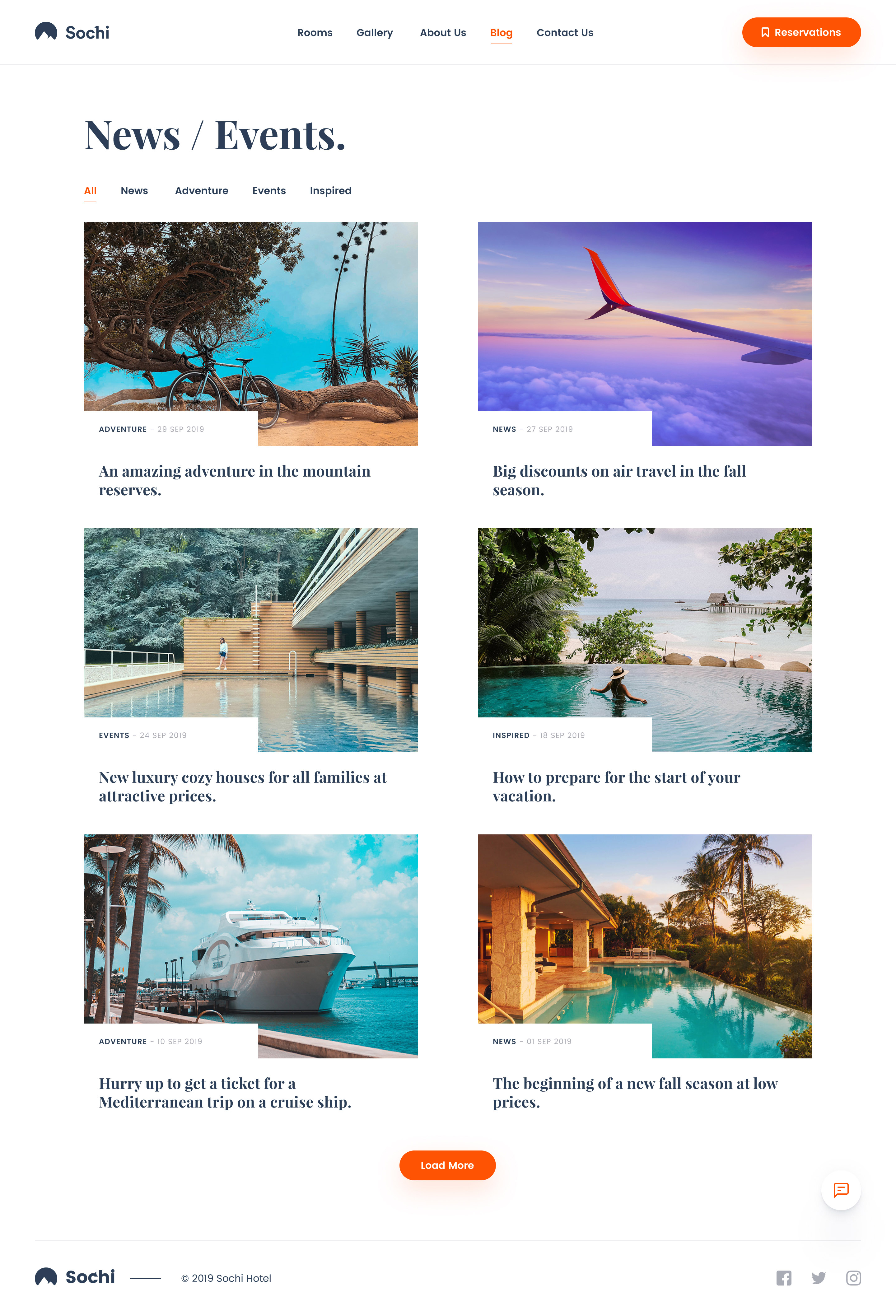This image is a screenshot taken from a mobile phone, depicting a webpage related to a location called "Sochi." The header features "Sochi" in the center, with a navy blue circular logo containing mountains in the background. Below the header, there is a navigation menu with options labeled "Rooms," "Gallery," "About Us," "Blog," and "Contact Us." The "Blog" option is currently selected, highlighted in orange with an orange underline.

On the far right of the header, there's an orange "Reservations" button with white text. The main content area below the menu is divided into sections showcasing news and events related to Sochi. 

Six prominent images are displayed in a grid layout, two per row, each paired with descriptive captions:

1. **Top Left:** "An Amazing Adventure in the Mountain Reserves" with an accompanying picture of the mountains.
2. **Top Right:** "Big Discounts on Air Travel in the Fall Season" featuring an image of an airplane.
3. **Middle Left:** "New, Luxury, Cozy Houses for All Families at Attractive Prices" accompanied by an image that includes a swimming pool.
4. **Middle Right:** "How to Prepare for the Start of Your Vacation" with another swimming pool image.
5. **Bottom Left and Right:** Two additional images with titles not specified, likely related to news and events.
   
At the bottom of the section, there is an orange "Learn More" button inviting further exploration.